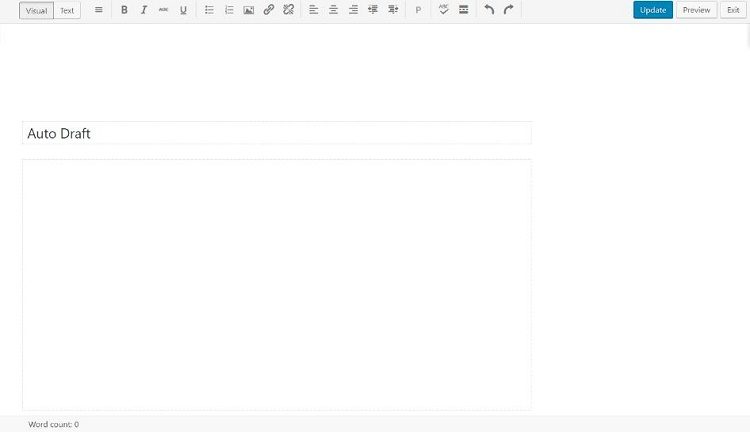The image is a horizontally rectangular screenshot of a data processing application, resembling Microsoft Word. The upper section of the frame features a banner of menus and icons. From left to right, the first menu is labeled "Visual" and is highlighted, followed by "Text." Next, there are various editing icons for formatting: Bold, Italics, Underline, Links, and Image, among others. Towards the right side of this top banner, there are three buttons—Update, Preview, and Exit—with the Update button highlighted in blue.

Beneath this top banner, there is a narrow horizontal field labeled "Auto-Draft," which appears to indicate an automatically saved draft. Below this, there is a larger blank rectangular text box area, ready for typing but currently empty. 

At the very bottom, a slender gray horizontal banner spans the full width of the image, displaying "Word count: 0" on its left side, indicating that there is no text in the document.